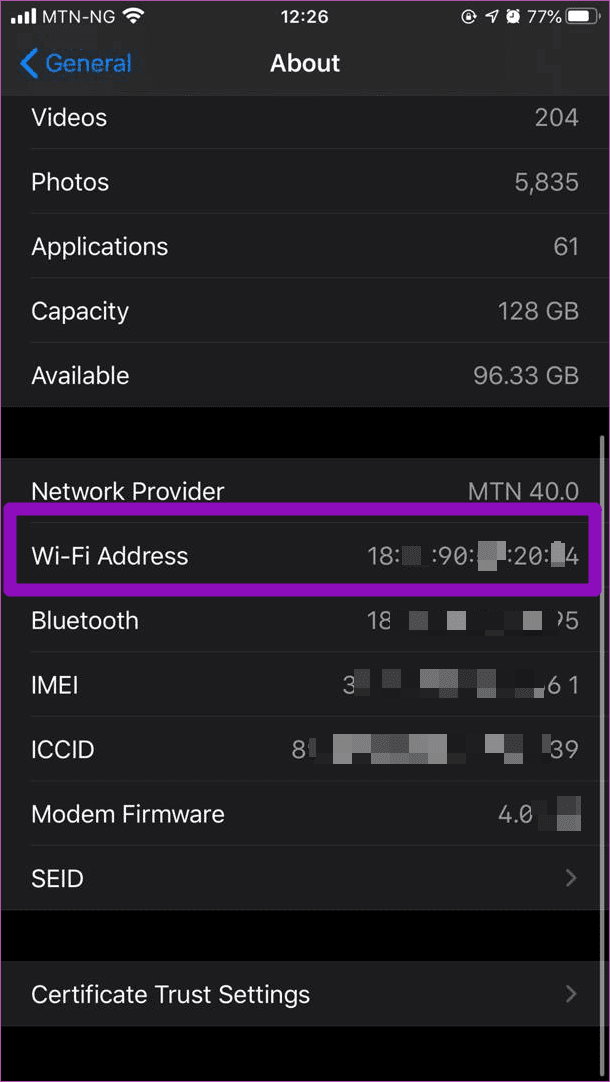The image features a smartphone screen with a predominantly black background. At the top of the screen, the status bar displays the network provider "MTN-NG," a WiFi icon, the time "12:20," a Telegram notification icon, and a battery level indicating "77%."

Centered at the top portion of the screen, the word "About" is prominently displayed. On the left side, there is a blue left-pointing arrow with the label "General" next to it.

Beneath "General," several statistics and details are listed in white text:
- "Videos" is accompanied by the number "204."
- "Photos" is accompanied by the number "5835."
- "Applications" is noted with the number "61."

Further down, storage information is displayed:
- "Capacity: 128 GB"
- "Available: 96.33 GB"

Below the storage details, additional device information is displayed, albeit partially obscured:
- "Network Provider: MTN 40.0"
- "WiFi Address:" mostly blurred but partially showing "18, 90, 20, and 4."
- "Bluetooth Address:" notably blurred, showing partial numbers "18 and 5."

On the left column of the screen towards the bottom, the terms "IMEI" and "ICCID" are listed, providing further device-specific identifiers.